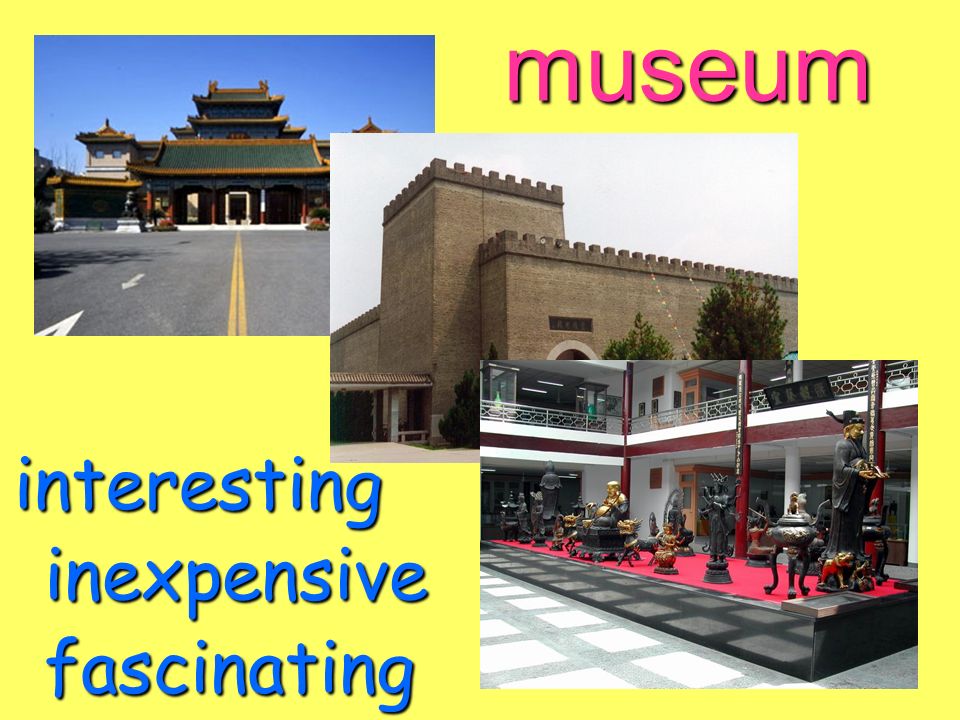The image is a vivid, bright yellow collage featuring three photographs, with the word "museum" written in hot pink lowercase letters in the top right corner and the words "interesting," "inexpensive," and "fascinating" in lowercase blue letters stacked in the bottom left corner. These words are written in a playful font and have a drop shadow.

The photographs are overlapped diagonally from the top left to the bottom right. The top left photo depicts the exterior of a traditional Asian-style building with multiple levels, resembling a pagoda, set against a clear blue sky. The middle photo features a castle-like structure, notable for its squared design and surrounded by trees, which imparts a majestic yet mysterious feel.

The bottom right photo showcases the interior of a museum, displaying a slightly raised platform draped in a red carpet and bordered by highly reflective black sides. On this platform stand various statues in black with gold accents, differing in size from medium to large, and exuding an aura of historical richness. The platform is situated beneath a visible balcony, adding to the depth and grandeur of the scene. Each of these photographs collectively captures the essence of culturally rich and visually intriguing museum exhibits.